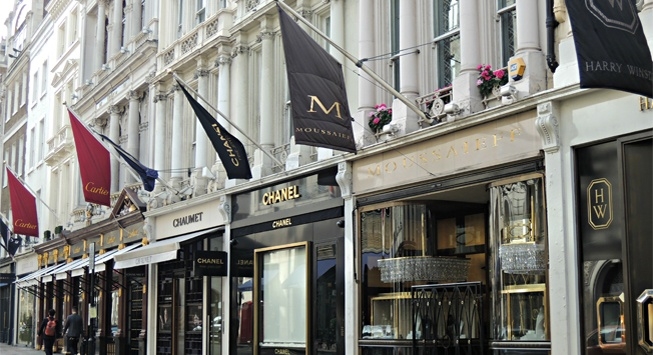The photograph captures an upscale strip mall during the daytime, featuring a series of high-end storefronts, including notable names like Chanel, Cartier, Harry Winston, and Mossor. The image is taken from a right angle, highlighting the architectural grandeur of the buildings, which showcase Roman-inspired white facades accented with gold trims, gold lettering, and glossy black walls. Above the chic storefronts, which all feature reflective glass displays, are two-story row homes characterized by their stone columns and Imperial aesthetic. Striking flags—some black and others red—protrude from the balconies of the second floor, amplifying the luxurious feel of the scene. The overarching structure appears to be four stories tall. The street scene is further animated by people walking near the Cartier store, enhancing the lively and sophisticated atmosphere of this high-end shopping district.